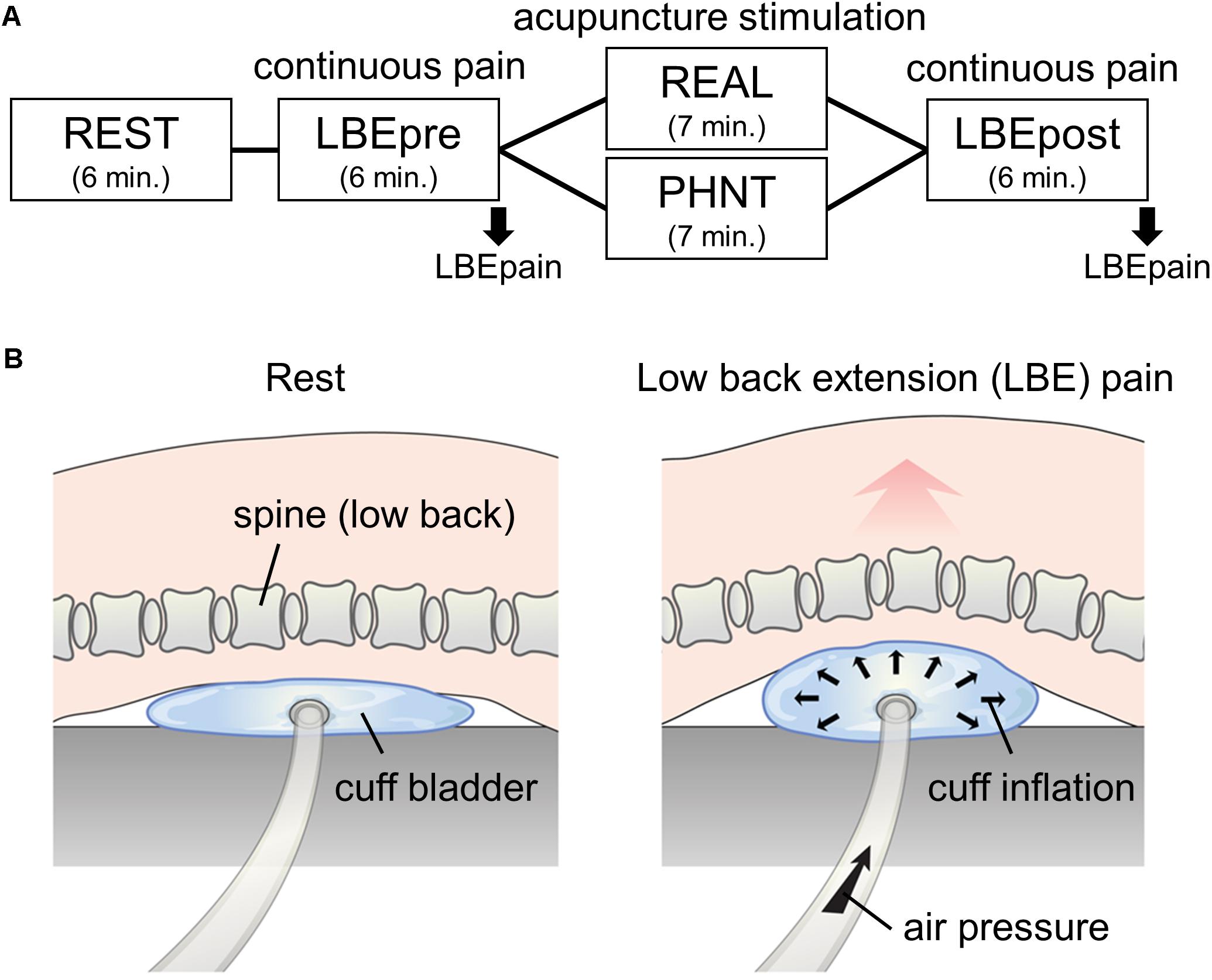This detailed image on acupuncture stimulation outlines a comprehensive protocol through both graphics and text. At the top, it specifies a sequence: rest for six minutes, continuous pain for six minutes, LBE (Low Back Extension) PRE for six minutes, acupuncture stimulation for seven minutes, PHNT (an unspecified term likely related to the treatment) for seven minutes, continuous pain, and finally LBE post for six minutes. Below this sequence, the image includes two diagrams. The left diagram features a pink background with an illustration of the spine marked "spine low back." It includes a blue "cuff bladder" below the spine, which is intended to be inflated to support and curve the spine during the LBE phase, potentially causing discomfort. The right diagram shows the same spine with the cuff bladder inflated, illustrating increased curvature and labeled as "cuff inflation air pressure," with arrows indicating airflow into the cuff. The left image notes "rest" above it, while the right notes "LBE pain." Together, these elements detail the step-by-step process for acupuncture stimulation and associated back support, emphasizing the sequence of rest, pain phases, and physical adjustments using the inflatable cuff.